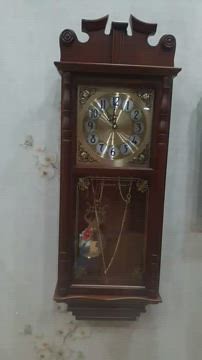The image showcases a rustic scene with a stone background that exhibits subtle gray tones on the right side. Dominating the center of the wall is a vintage wooden clock, crafted from rich brown wood. The clock features ornate shapes at the top, and the clock face itself is made of brass metal, displaying numerals from 1 to 12. The hands of the clock point to the four cardinal directions: top left, top right, bottom left, and bottom right. Reflective light glints off the middle of the clock face, adding a touch of luminosity. Below the clock, there is a window, and suspended from the clock is a brown metal pendulum, positioned centrally. The edges of the clock are adorned with colors, and the bottom lip of the clock shows some intricate detailing. The stone wall also has visible cracks, lending an air of antiquity and character to the scene.